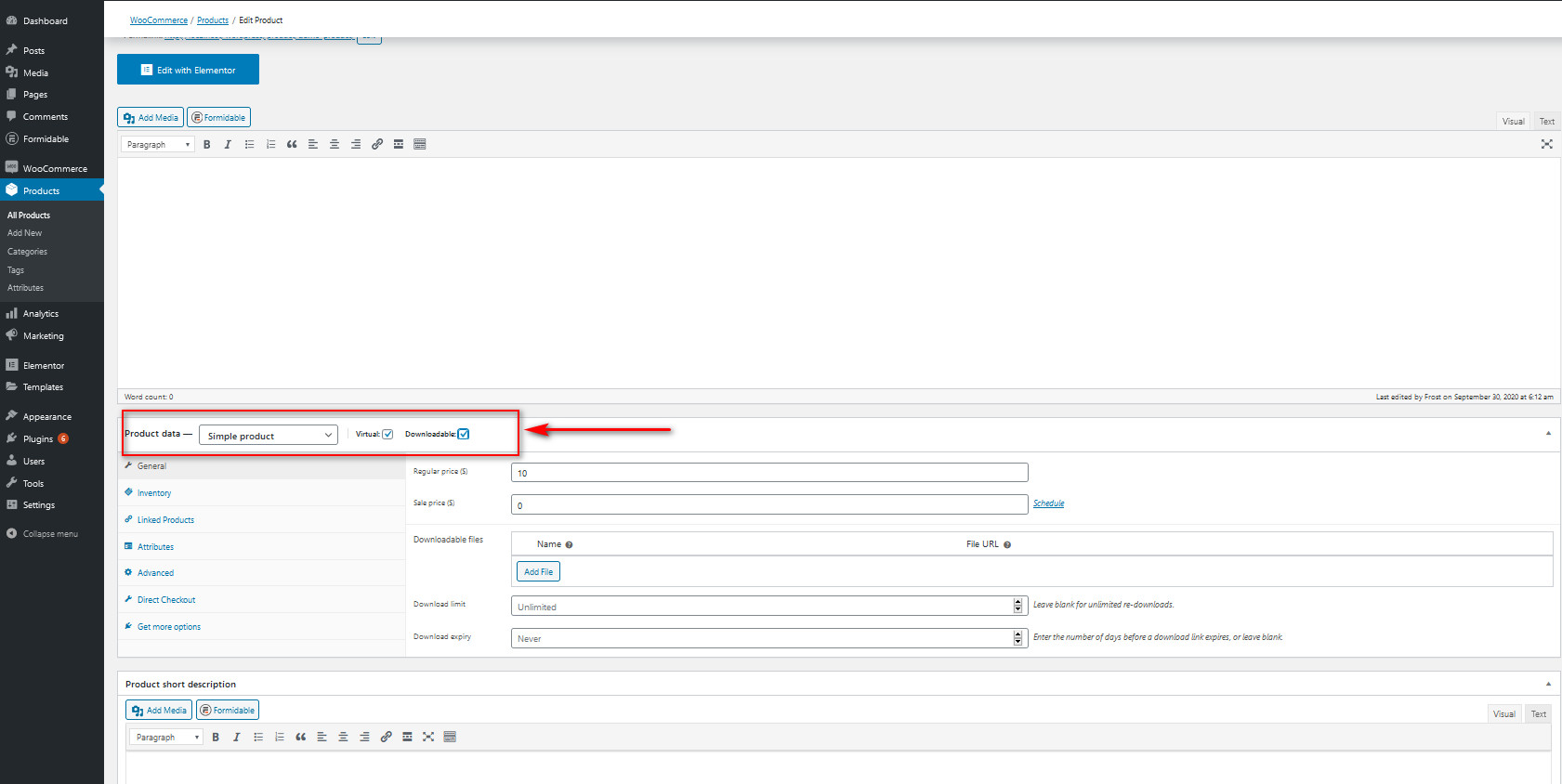The image depicts a complex, tech-oriented interface on a large screen. The left pane features a black background with white text, highlighted on the "Products" section of an apparent dashboard. Other navigational items like "Appearance" and "Settings" are partially discernible. The main section on the right consists of a spacious white area intended for text input, though the specific use is unclear due to the small, hard-to-read text. Below this primary text field, there are additional formatting options including italics, bold, paragraph separation, and quotations, indicating that the interface supports sophisticated text editing. The overall design suggests the interface is used for a technical application, possibly related to network management, IT, or software development.